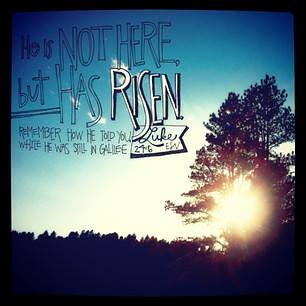An evocative image captures the serene moment of dawn or dusk, where the light of the setting or rising sun shines brilliantly through the silhouette of shadowy pine trees positioned on the right. The sky transitions from a light hue at the horizon to a slightly darker shade towards the top, adorned with scattered clouds. The entire foreground is rendered in deep black due to an out-of-focus forest brush that stretches across the bottom of the image. 

On the upper left, overlaying the sky, an inspirational Christian quote is prominently displayed in a handwritten-like font, bordered by a thin black outline. The text reads: "He is not here, but has risen. Remember how he told you while he was still in Galilee." Beneath this message, there is a Bible reference, "Luke 24:6," followed by "EN," which seems to denote a version number. The composition and elements suggest this image may serve as an advertisement or message for a church, especially pertinent around Easter but suitable for any time of the year. The overall color palette is dominated by hues of white, blue, and black, enhancing the spiritual and serene atmosphere of the scene.